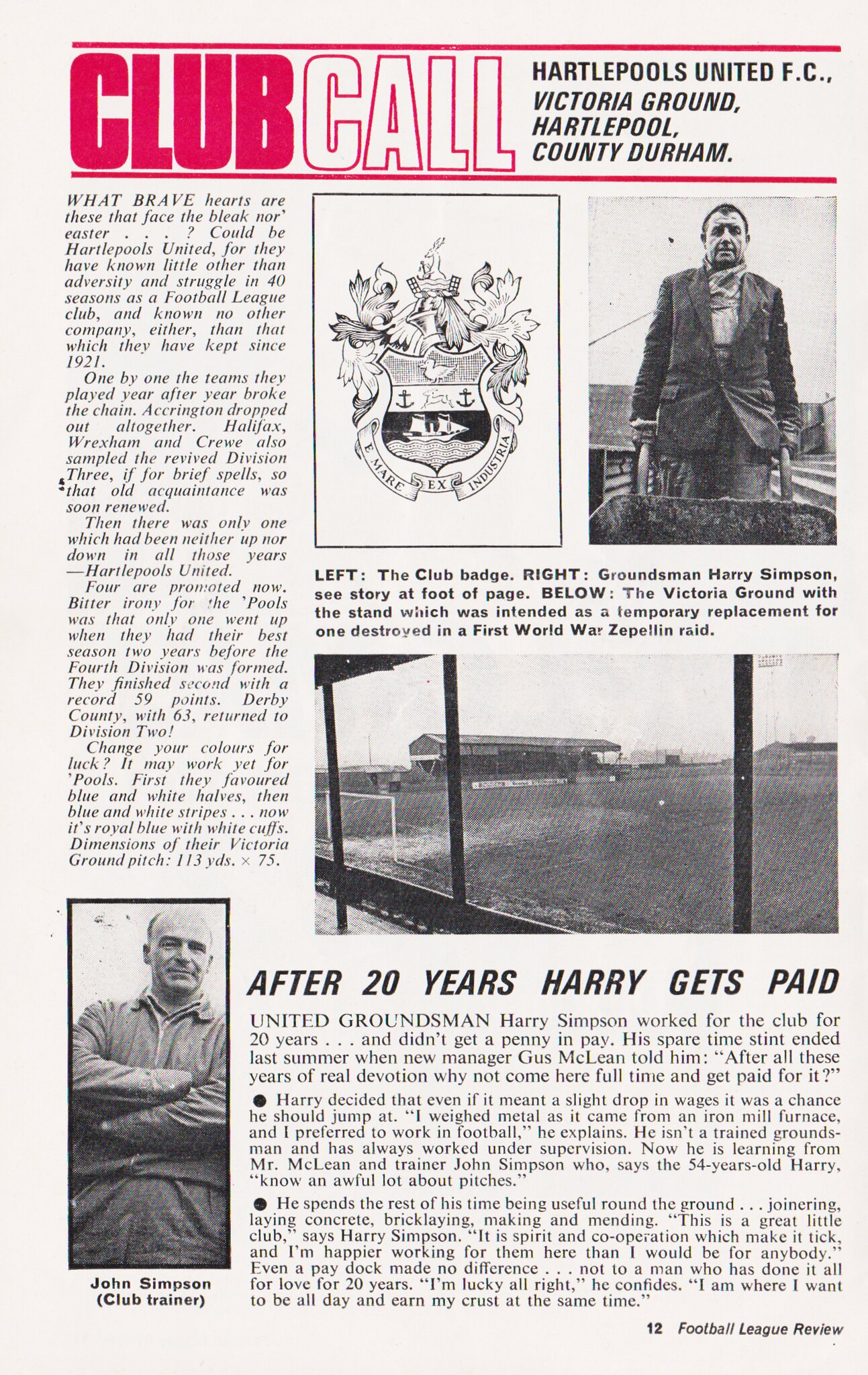This image depicts an excerpt from an old football program, characterized by its off-white color and black-and-white photographs. The top of the page prominently features a title in big block letters, with "Club" filled in red and "Call" outlined in red, all within a red rectangular box. To the right of the title, in smaller black text, it reads: "Hartlepool's United FC, Victoria Ground, Hartlepool County, Durham."

Below the title, the left-hand side of the page contains several paragraphs of text, forming an article. To the right of the text, occupying the center and right sections, are two images. One image is of a crest resembling a shield with decorative elements. Below this, there is a black-and-white photograph of a man in a suit pushing a wheelbarrow, facing the viewer. Further down, in the bottom right corner, another image shows a man with his arms folded across his chest; he is balding and middle-aged. Next to him is text that reads: "John Simpson (Club Trainer)." 

Additionally, another picture in the middle right section of the page shows a view looking out onto a field. The page number at the bottom right indicates that this is page 12 from the "Football League Review." An additional header at the bottom mentions: "After 20 years, Harry gets paid." This detailed layout and imagery encapsulate a significant historical snapshot of Hartlepool United FC.